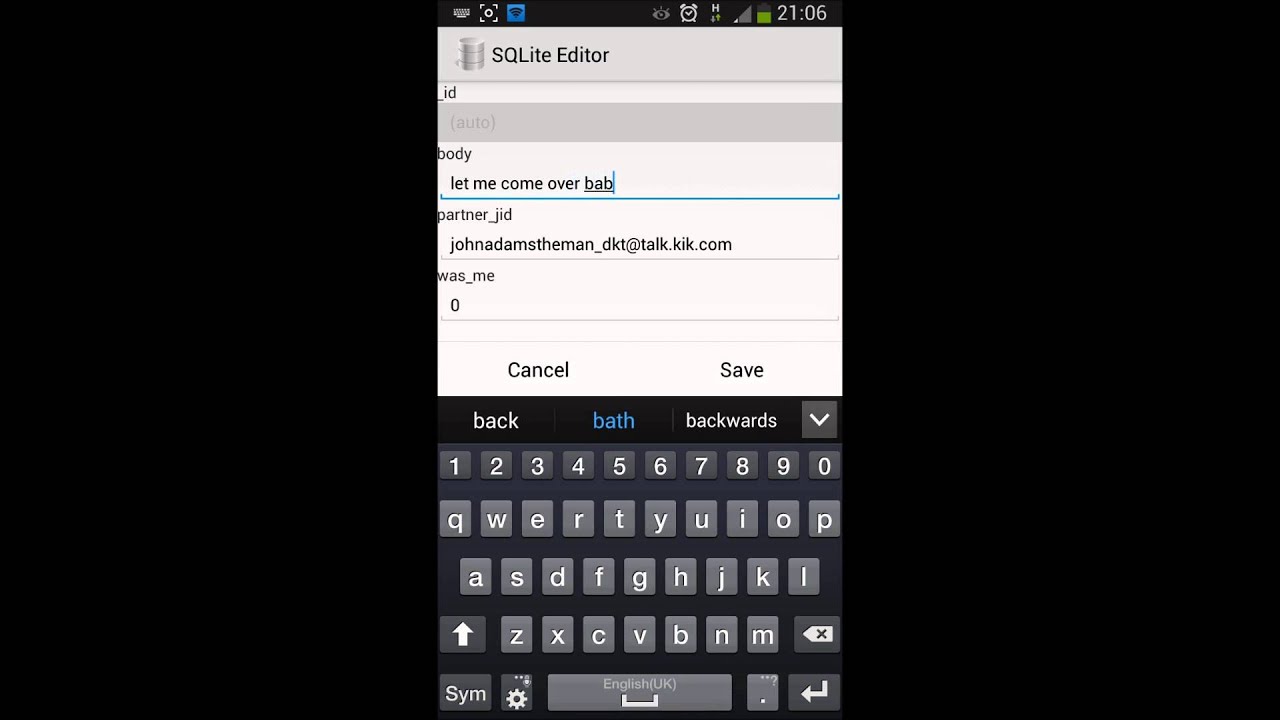This landscape-mode screenshot prominently features a smartphone screen capture at its center. The smartphone display showcases an application with a predominantly white interface. At the top of the screenshot, a series of standard smartphone icons are visible, indicating elements such as signal strength, battery status, and notifications.

Beneath these icons, the text "SQLite Editor" is clearly displayed, followed by the label "ID," both set against the white background. A horizontal gray banner separates this section from the next, which is designated as "Body." Here, multiple lines of text on a white backdrop can be observed:

- "Let me come over"
- "Babe"
- "partner under_bar JID John Adams"
- "the man under_bar DKT at talk.kik.com"
- "was under_bar me zero cancel and save"

At the bottom of the screenshot, a virtual keyboard is visible, suggesting predictive text options such as "back," "bath," and "backwards." The entire framing on the left and right sides of the screenshot is black, emphasizing the central focus on the smartphone display.